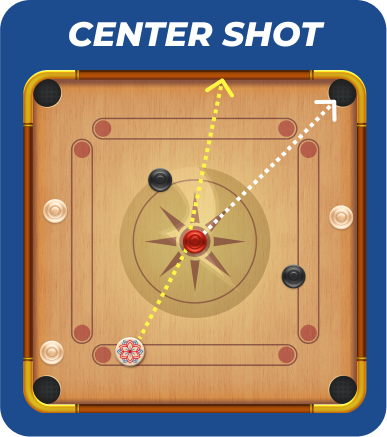The image is a digitally enhanced, full-color photograph with a vertically rectangular shape and rounded corners against a solid blue background. The top of the image features the word "CENTERSHOT" in all capital letters, rendered in white text. The focal point of the image is a square wooden game board, reminiscent of a mix between billiards and shuffleboard. This game board includes corner pockets and a central star-shaped marking. 

On the game board, players use checker-like pieces, with black and red disks positioned strategically, and a noticeable white disk used to make shots. The white disk appears to act as the equivalent of a pool cue ball, designed to knock the other disks into the corner pockets. The image combines elements of various traditional games, illustrated with arrows to indicate potential shot trajectories. The scene has no people depicted, focusing solely on the game setup.